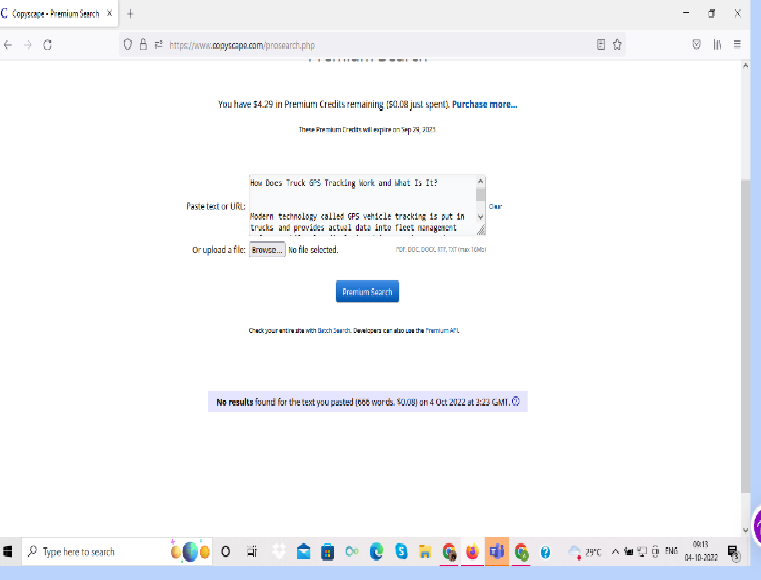**Screenshot of an Unreadable Browser Page**

This image showcases a screenshot of a browser page where the textual content is too blurry to discern. The majority of the text is displayed in black, with certain segments highlighted in blue. A prominent blue button is visible on the page. At the bottom of the screenshot, there is a collection of pixelated symbols alongside a search bar, likely part of the browser's user interface.